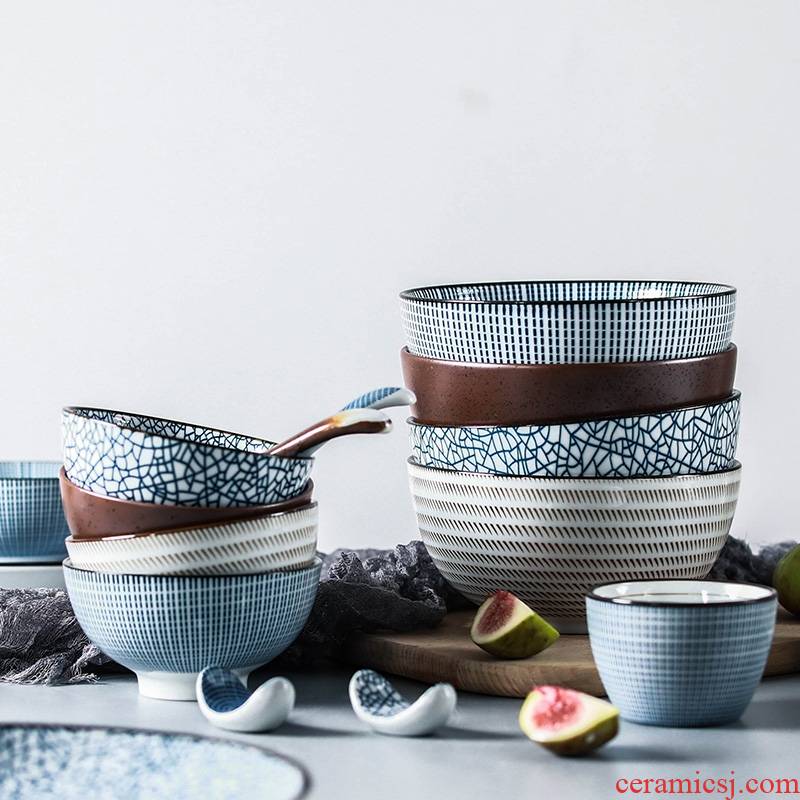The photograph showcases a meticulously arranged collection of ceramics, predominantly featuring stacked bowls in various sizes and designs. There are four medium white bowls with intricate blue or silver patterns, including dashed lines and plaid-like textures, nested within each other. To their right, a similar set of four larger bowls also displays these detailed designs, but one medium and one large bowl stand out with a dark metallic brown sheen. Nestled among these collections, a smaller cup appears in the foreground, mirrored by another in the background.

On the table, which doubles as a counter, a rustic wooden board supports the larger bowls and one piece of realistic fruit design—a possible kiwi with a green peel and pink seeds. The table surface also features two segments of ceramic fruit and a mixture of ceramics and what appear to be rocks. Notably, an arrangement resembling a lazy Susan holds additional bowls. The top medium bowl intriguingly contains two spoons—one with a brown handle and another featuring blue and white stripes—sticking out.

The overall color palette of the ceramics is primarily white with blue, brown, and silver accents, while black, gray, and whitish-blue tones form the background, adding a subtle, cohesive aesthetic. The lower right corner of the image features a red font inscription, "ceramicsj.com," hinting at a possible advertisement. The setting, adorned with a mix of ceramic pieces and realistic fruit designs, evokes both elegance and functionality in a cohesive set.